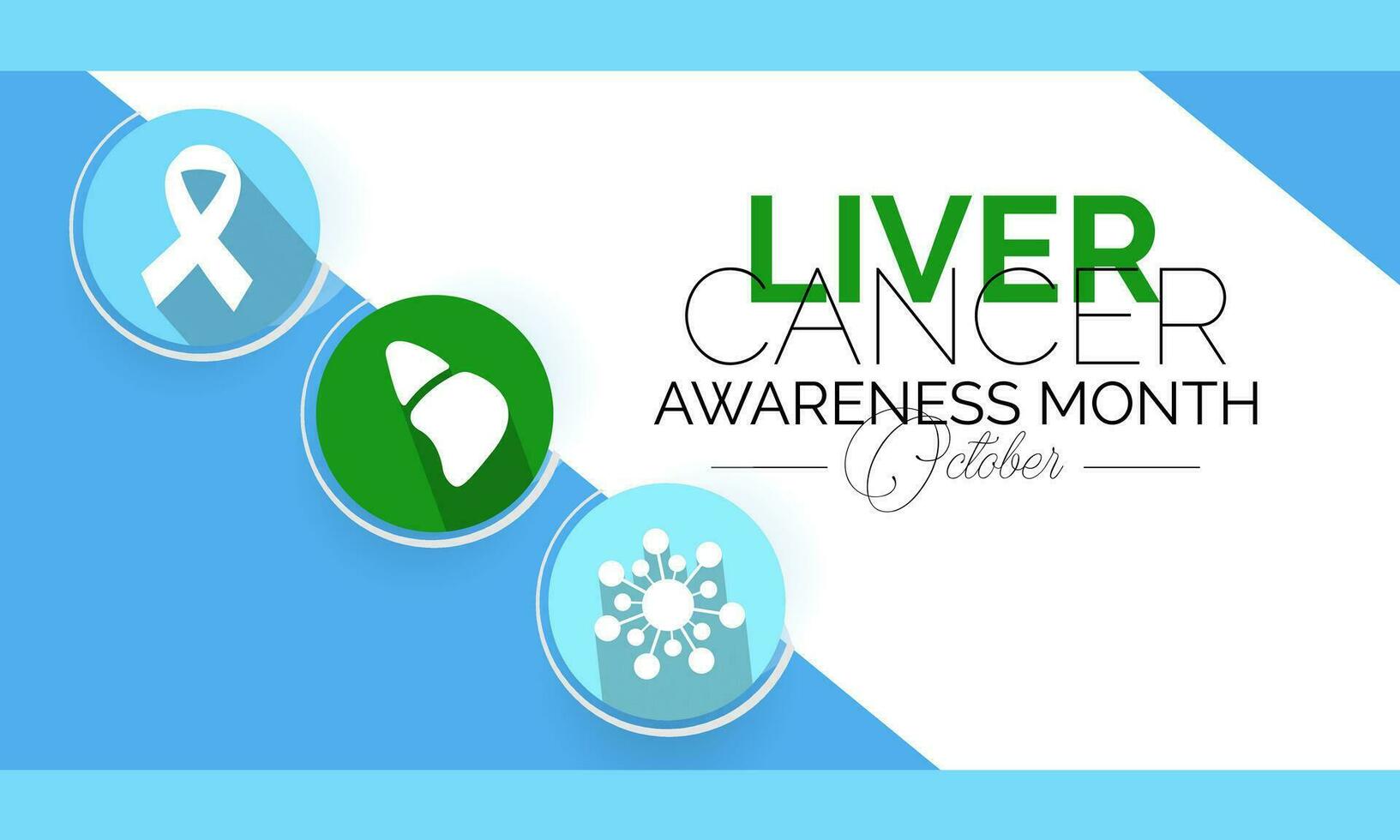The image is a digital advertisement for Liver Cancer Awareness Month in October, predominantly featuring shades of blue. A light blue band runs across the top and bottom of the rectangular image, framing the central elements. The focal point includes a vertical arrangement of three cascading circles starting from the top left. The first circle is light blue, showcasing a white silhouette of an awareness ribbon. Below and slightly to the right of it is a green circle with a white silhouette resembling the shape of a liver. Further down is a lighter blue circle displaying a white, intricate design that resembles a snowflake or a molecular structure. The prominent text "Liver" appears in green, "Cancer" in a thin black font, and "Awareness Month" in matching black. The word "October" is written in a cursive hand font. The overall design integrates a clean, blue and white aesthetic with clear, specific imagery relevant to liver cancer awareness.